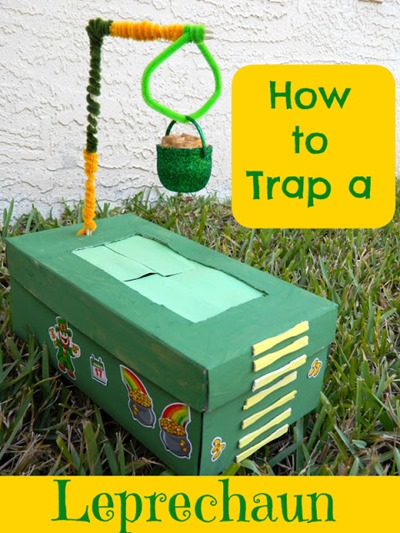The image captures a humorous, handmade leprechaun trap crafted from a green shoebox, positioned diagonally on a patch of short, St. Augustine grass. The backdrop features a white, even-textured wall. The shoebox is meticulously colored green with a light green rectangular cutout on the top, partially covered by slitted blue paper designed to mimic a trap door.

Atop the shoebox is an elaborate setup involving a yellow and green coiled stem with a secondary perpendicular stem acting as a holder. From this holder, an inverted L-shaped structure suspends a green bucket filled with brown objects, resembling gold or rocks. This setup is part of the imagined mechanism to lure and trap a leprechaun.

The shoebox is adorned with various thematic stickers. The right side features a crown, a calendar with the number 17, a rainbow, and a jar of fruit, while other sides display a leprechaun alongside pots of gold with rainbows. Frontally, the box displays seven yellow, horizontal-lined segments, adding to its decorative aspect.

To the left side of the image, text reads "How to trap a leprechaun" in green letters against a yellow background. The word "leprechaun" also appears at the bottom within a yellow rectangular frame. This playful creation suggests that a leprechaun would be enticed by the faux gold, only to get trapped inside the shoebox.